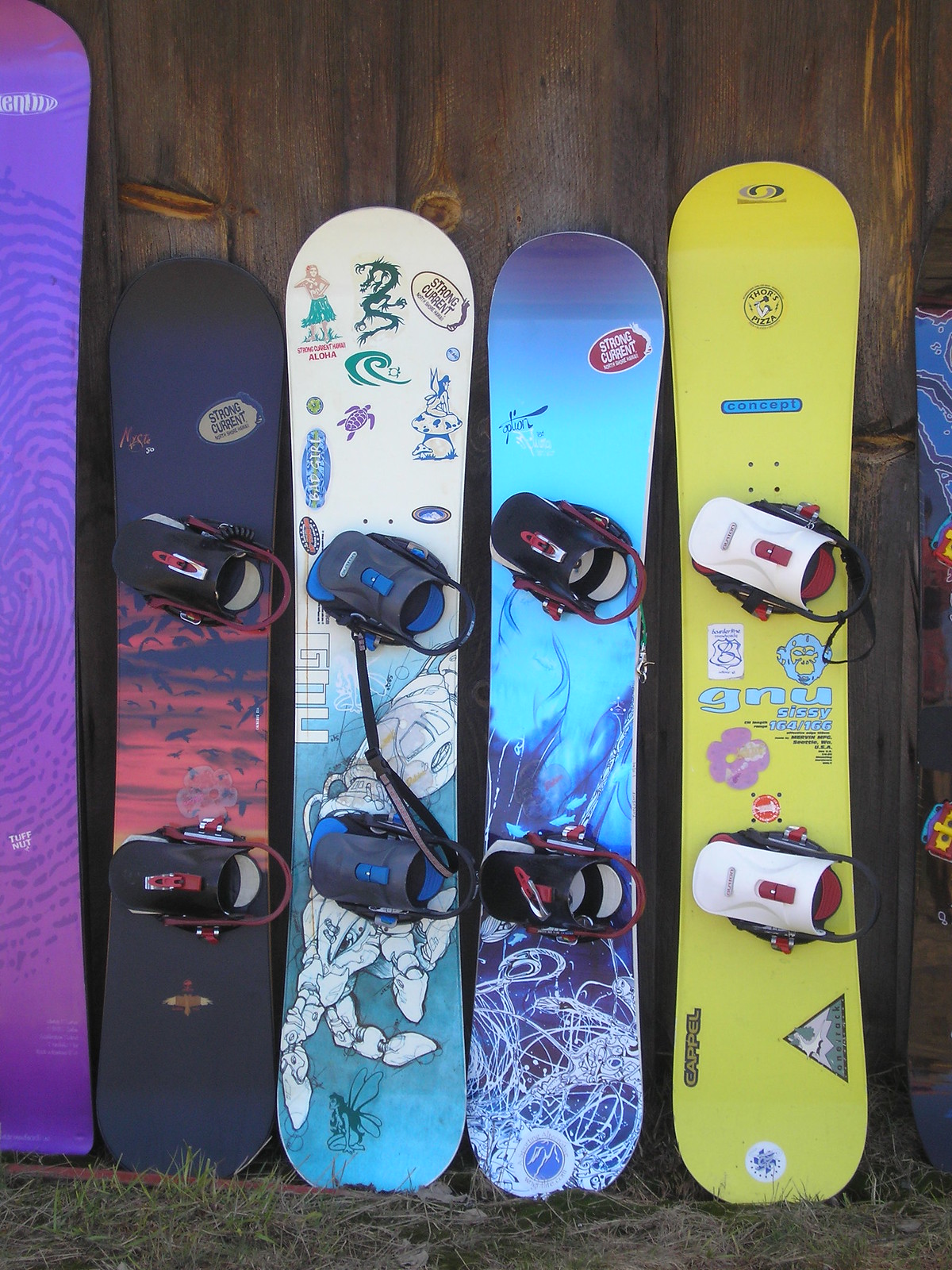This detailed photograph depicts a series of five snowboards leaning against a dark brown wooden wall, likely the side of a cabin. The boards are arranged in a row on grass, with no snow visible, suggesting they are used and possibly for rent at a ski resort. Each snowboard is distinct in color, design, and size, providing striking visual variety.

From left to right:

1. **Purple Snowboard**: The tallest in the lineup, with a unique fingerprint design.
2. **Black Snowboard**: Featuring a dark night scene with a red sky and ravens flying through it.
3. **White Snowboard**: Adorned with a cyborg arm and a combination of blue and white colors, it also sports several stickers, including "Strong Current".
4. **Blue Snowboard**: Displaying a water-themed design with blue and white swirls and an artist's signature.
5. **Yellow Snowboard**: The rightmost board is banana yellow, covered in various logos and designs, including a gorilla, flowers, and the words "GNU" and "Thor's Pizza."

The image suggests these snowboards are possibly for children, indicated by their relatively small footholds. The scene blends a rustic backdrop with vibrant, creative snowboard designs, highlighting both the practical and artistic elements of winter sports equipment.